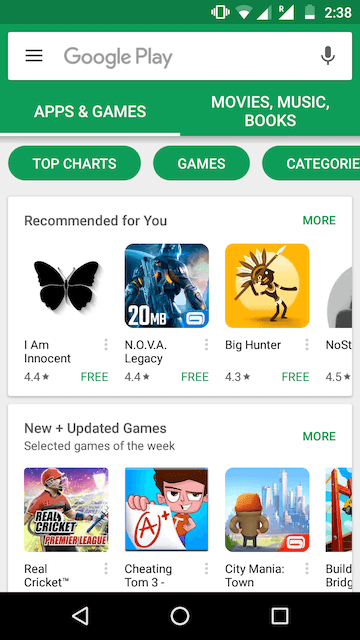The image displays a Google Play Store interface with a white background, showcasing a variety of applications. Eight applications are partially visible, with six fully shown and two on the right side partially cut off. The top part of the image features a green background with five white text labels: "Apps & Games," "Movies," "Music," and "Books." Above these tabs is a white search box displaying "Google Play."

Below the green tab section, there are white filter buttons with green text, such as "Top Charts" and "Games Category." Under these buttons, a section titled "Recommended for You" displays several free games. "I'm Innocent" is listed, although no further details are given. "Nova Legacy" by Gameloft, which is 20 megabytes and rated 4.4, is shown next. Another featured game is "Big Hunter," rated 4.3 and also free, depicted with an image of a hunter holding a spear against a yellow sunset background. The last visible app in this row is rated 4.5, but its name is not shown.

At the bottom, there’s a section titled "New + Updated Games" and "Selected Games of the Week." It includes "Real Cricket," illustrated with an image of a person playing cricket. "Cheating Tom 3" shows a character named Tom holding a paper marked with an "A+" in red text. "City Mania" features an image of a person observing a city, created by Gameloft, indicated by a "G" in the bottom right corner. The last application in this section is "Build Bridge," but it is only partially visible.